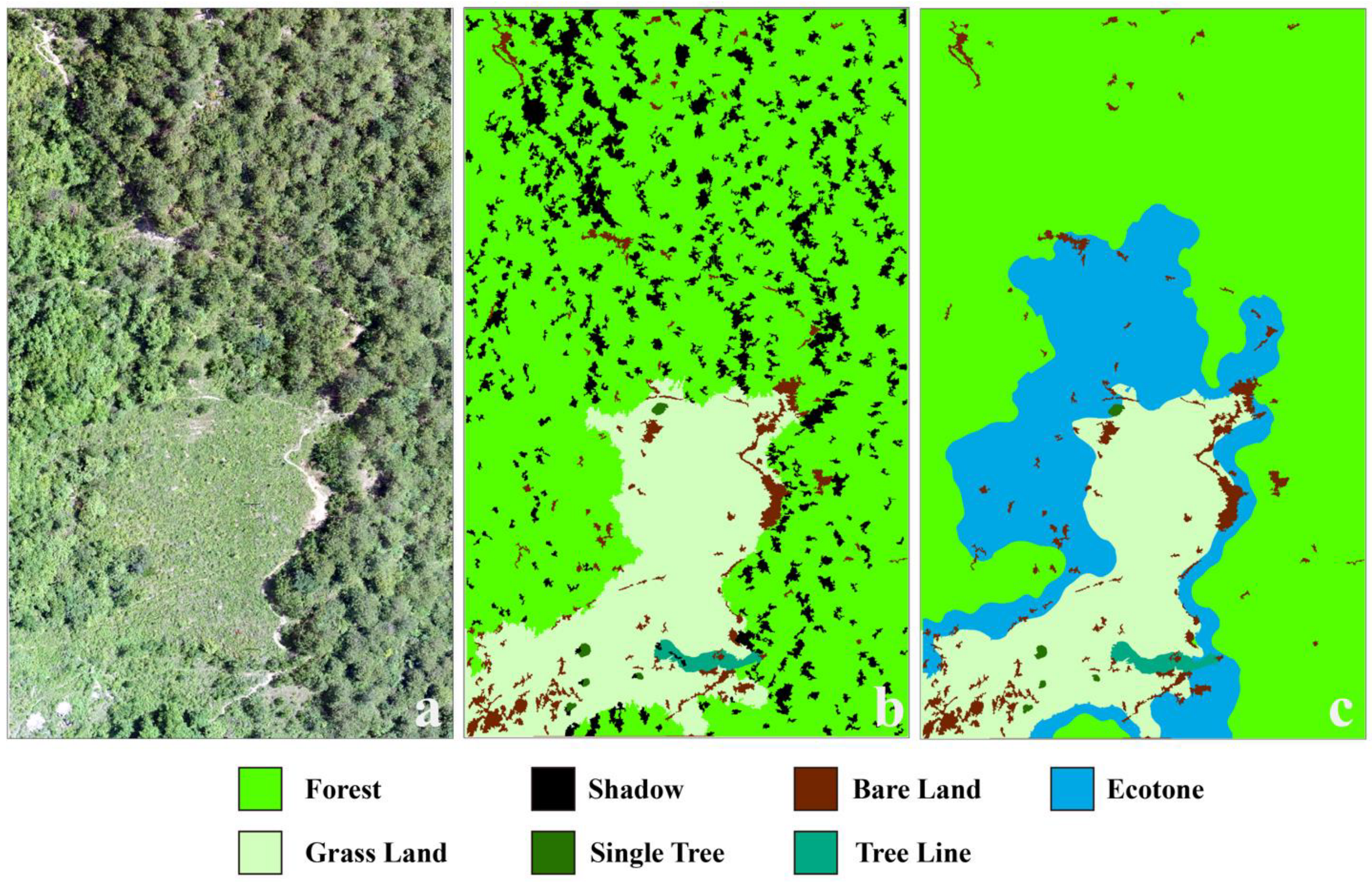The image consists of three rectangular panels side by side, each depicting a different representation of the same geographic area. The leftmost panel, labeled A, is a realistic aerial photograph showing a lush, green forest with a meadow area visible in the bottom left corner. This section is characterized by fewer trees and a vibrant, green expanse.

The middle panel, labeled B, presents a less realistic, more artistic rendition of the same area. Here, the trees are depicted in bright neon green with black shadows interspersed, while the meadow is a mix of lighter greens, almost yellow, with red tones. This panel also highlights a mountain range within the region.

The rightmost panel, labeled C, simplifies the landscape further with broad, abstract representations. The forest is shown in neon green, the shadowed areas in black, and the meadow in a mix of yellow and red hues. Additionally, there are blue patches representing ecotone zones and a blend of colors for various terrain features.

Below the panels, a comprehensive key explains the color coding: bright green for forest, black for shadow, dark red (or maroon) for bare land, light blue for ecotone, light green for grassland, dark green for single tree, and a bluish-green for the tree line.